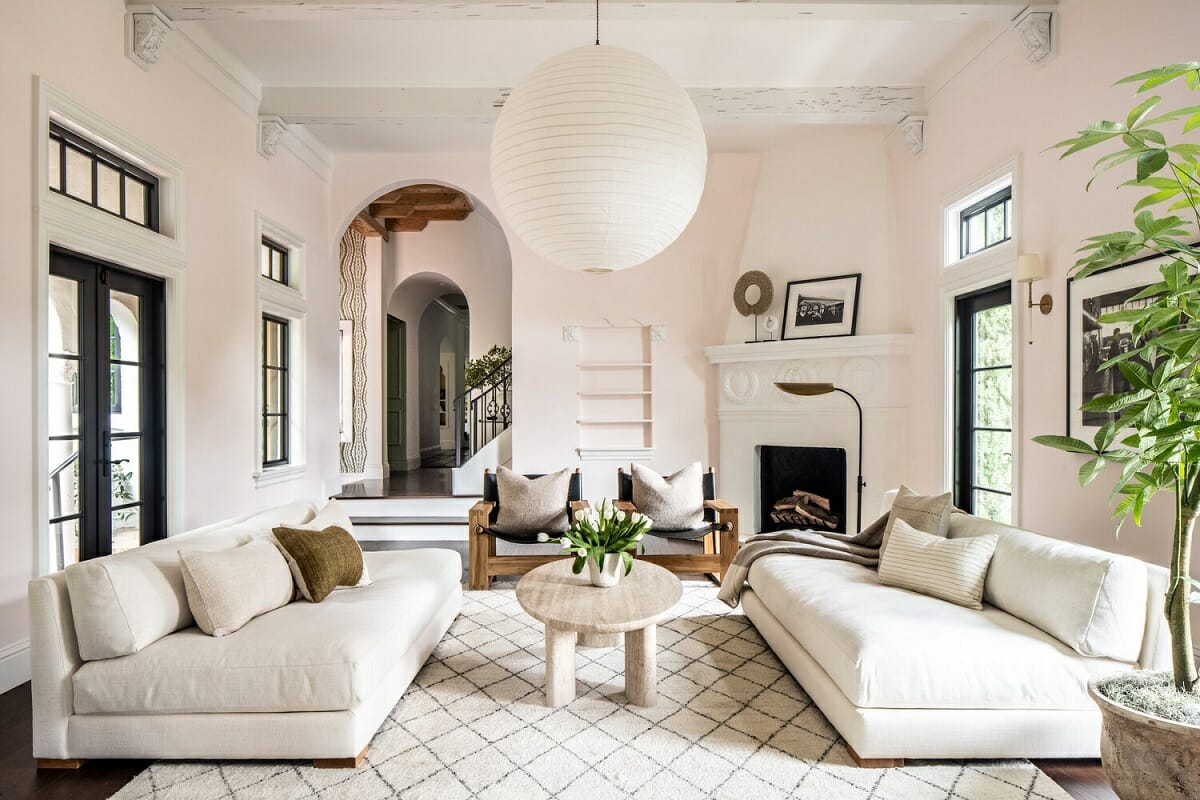This image is an interior view of a tastefully designed living room, captured as a 3D color rendering illustration in landscape orientation, likely created with an app like SketchUp. The room portrays an elegant and serene ambiance with predominantly white and pale pink hues.

The room features very pale pink walls, accented with white outlines around the doors and windows. On the left, there are double doors with transom windows, while on the right, a black-framed window adds contrast. The focal point of the space includes two low white sofas with upholstered pillow backs and several toss pillows, symmetrically placed on the left and right sides of the room. Additionally, a white rug with a gray crisscross diamond pattern is laid beneath both sofas, enhancing the room's cohesive look.

Central to the room is an oval light brown coffee table with a beige marble finish and short legs, adorned with a white vase holding white tulips. This coffee table sits on a white rug with a crisscross diamond pattern, complementing the room's light and airy color scheme. The back wall features built-in shelves next to a white, angled fireplace, while an indented bookcase stands empty in the middle.

There are several architectural features that add depth to the room, including an arched entryway to the left, leading to a staircase partially visible behind it. Above the living area, a large, circular white globe pendant light, resembling a rice paper lantern, hangs suspended from the ceiling, completing the room's cohesive and elegant design. The overall effect is a bright, welcoming space with a harmonious blend of modern and classic elements.